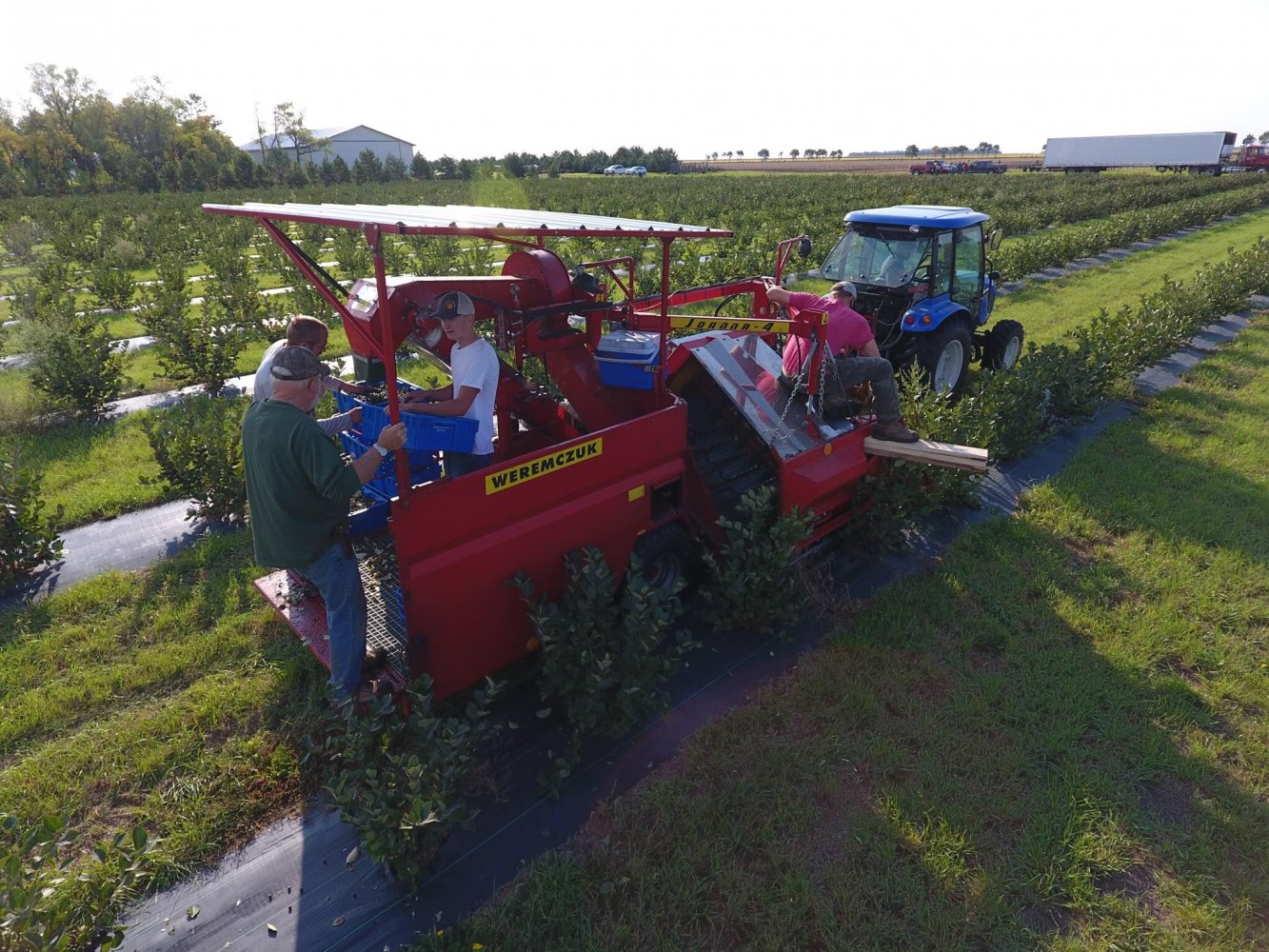The photo captures a bustling farm scene during harvest time, featuring rows of bushy plants that closely resemble blueberries, with a layer of black plastic underneath and wide rows between them. Central to the scene is a blue tractor with an enclosed cab, having smaller front wheels and larger rear wheels, which is towing a red harvester machine adorned with the text "WEREMCZUK" in yellow and white. The harvester's structure includes a slanted roof and is actively engaged in picking the berries. At the front of the harvester, a young man in a ball cap directs the plants into the machine, while the picked berries travel up a ramp through a divider to be packed into crates. On the back platform, another young man in a green shirt, blue jeans, and a gray baseball cap with a wristwatch on his left arm, appears to be overseeing the process. A second small red tractor can be seen behind the harvester, both facing to the right amidst the lush green agricultural field. The distance reveals some barns, parked vehicles, and expansive open fields extending to the horizon, highlighting the picturesque and industrious atmosphere of the farm.